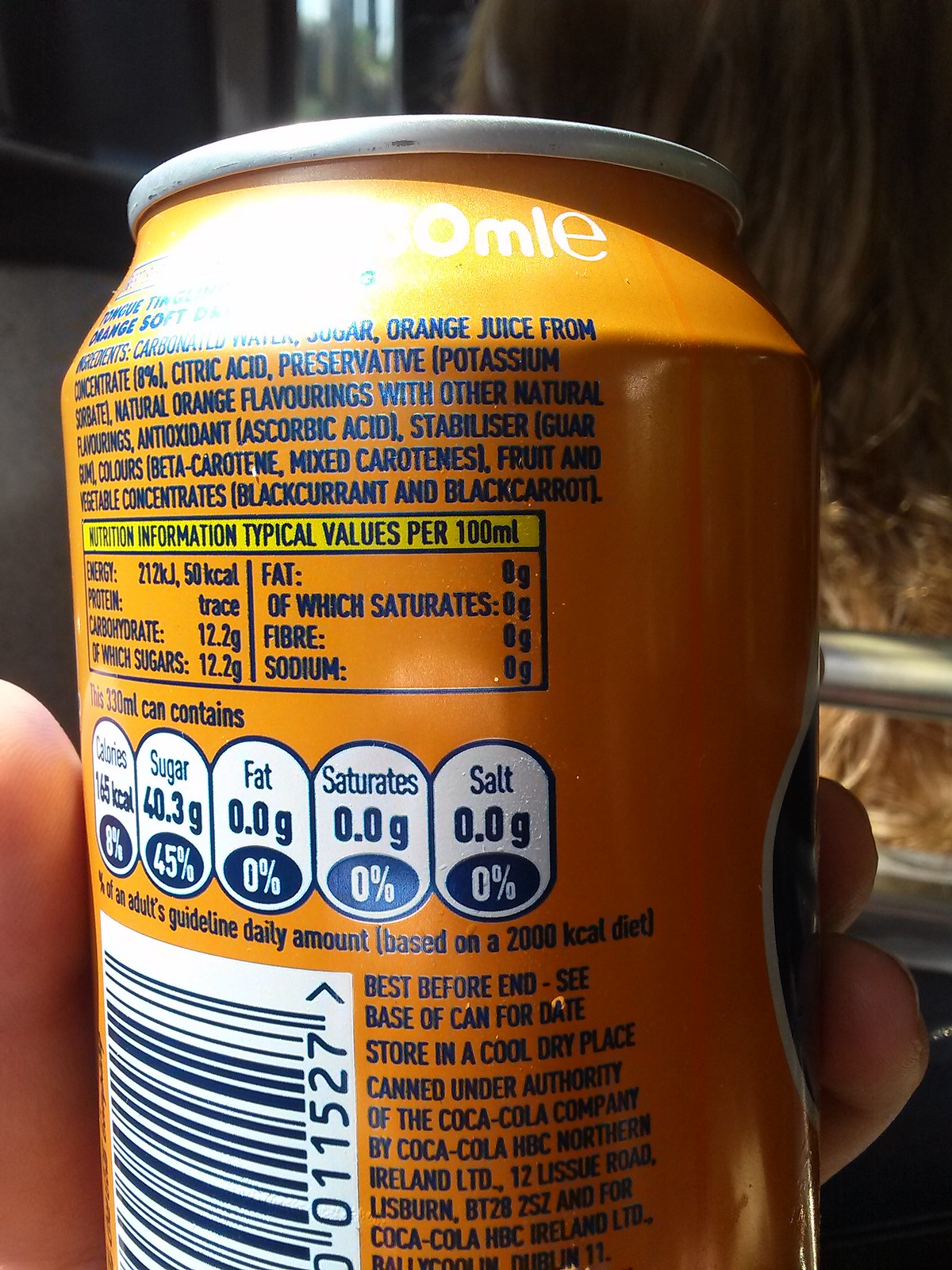This is a detailed color photograph capturing a close-up of a drink can held by a person's fingers. The image focuses on the back of the can, revealing a portion of an ingredients list and nutritional information table. The can's top edge is grey, and its body is predominantly orange, adorned with black text. The left edge of the can is partially obscured by one finger, while two more fingers are visible along the right edge. 

The blurred section towards the top, caused by light glare, obscures some of the text. Below the black text, the nutritional contents table lists values for fat, fiber, sodium, and other elements. Further down, the can displays information about the amounts of sugar, fat, saturates, and salt, along with their corresponding daily allowance percentages, which are situated within white ovals with black text.

On the lower left-hand corner of the can, a black barcode set against a white background is visible, alongside a best-before date that is partially obscured. The background of the photograph is predominantly dark, with a window at the top contributing a hint of ambient light. Two silver bars are positioned to the right, partially concealing beige objects behind them.